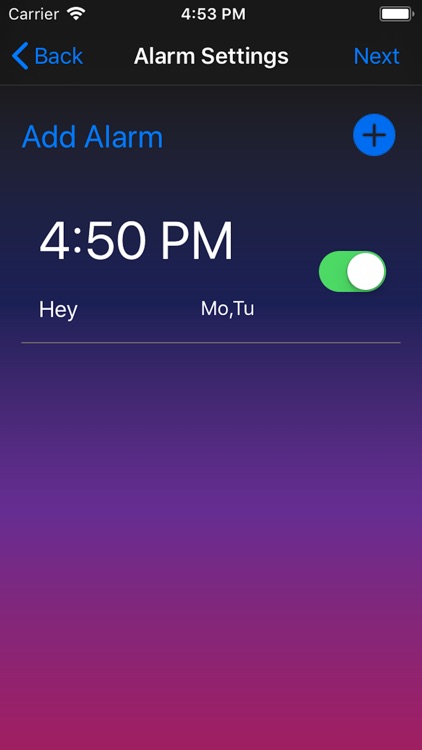This image is a screenshot from a smartphone. At the top, the background is black. On the left side in white font, it says "Carrier," followed by the Wi-Fi icon. In the middle, the time is displayed as "4:53 PM." On the right side, the battery icon appears to be almost fully charged.

Beneath the time, in bold white font, it reads "Alarm Settings." To the left of this text, there's a blue "Back" option with an arrow pointing left. On the right side, in blue, it says "Next." Below this, in blue font, it reads "Add Alarm" and on the right side of this text, there is a blue circle with a black plus sign in it.

The background color starts to gradually lighten from this point. It transitions from a dark purple to a lighter purple, almost lavender hue. At the very bottom, the background changes to a deep pink or very dark pink color.

In the top third of the screen, beneath the "Add Alarm" section, there's a large white font displaying "4:50 PM." Below this, in smaller white font, it says "Hey." In the center, abbreviations "MO" and "TU" are visible, indicating Monday and Tuesday. To the right of the "4:50 PM" time, there's a white circle, and to the left of this, a green indicator, showing that the alarm is turned on.